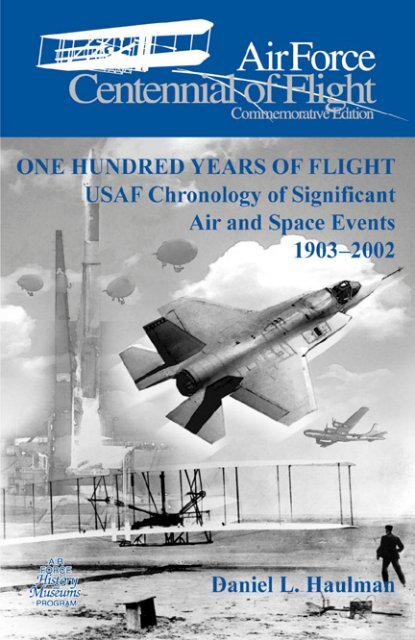The image is a vintage-style cover of a book or magazine titled "Air Force Centennial of Flight Commemorative Edition," with a blue banner at the top featuring a white plane design. The subtitle reads, "100 Years of Flight: USAF Chronology of Significant Air and Space Events, 1903-2002." The cover includes a black-and-white collage of various aerial vehicles, including old and modern planes, blimps, spacecraft, and a rocket system. Prominently featured is the original Wright Brothers plane, and a man is seen standing on the ground in the foreground. The author, Daniel L. Hallman, is credited in blue text on the bottom right. Additionally, the bottom left corner mentions the "Air Force History Museums Program."